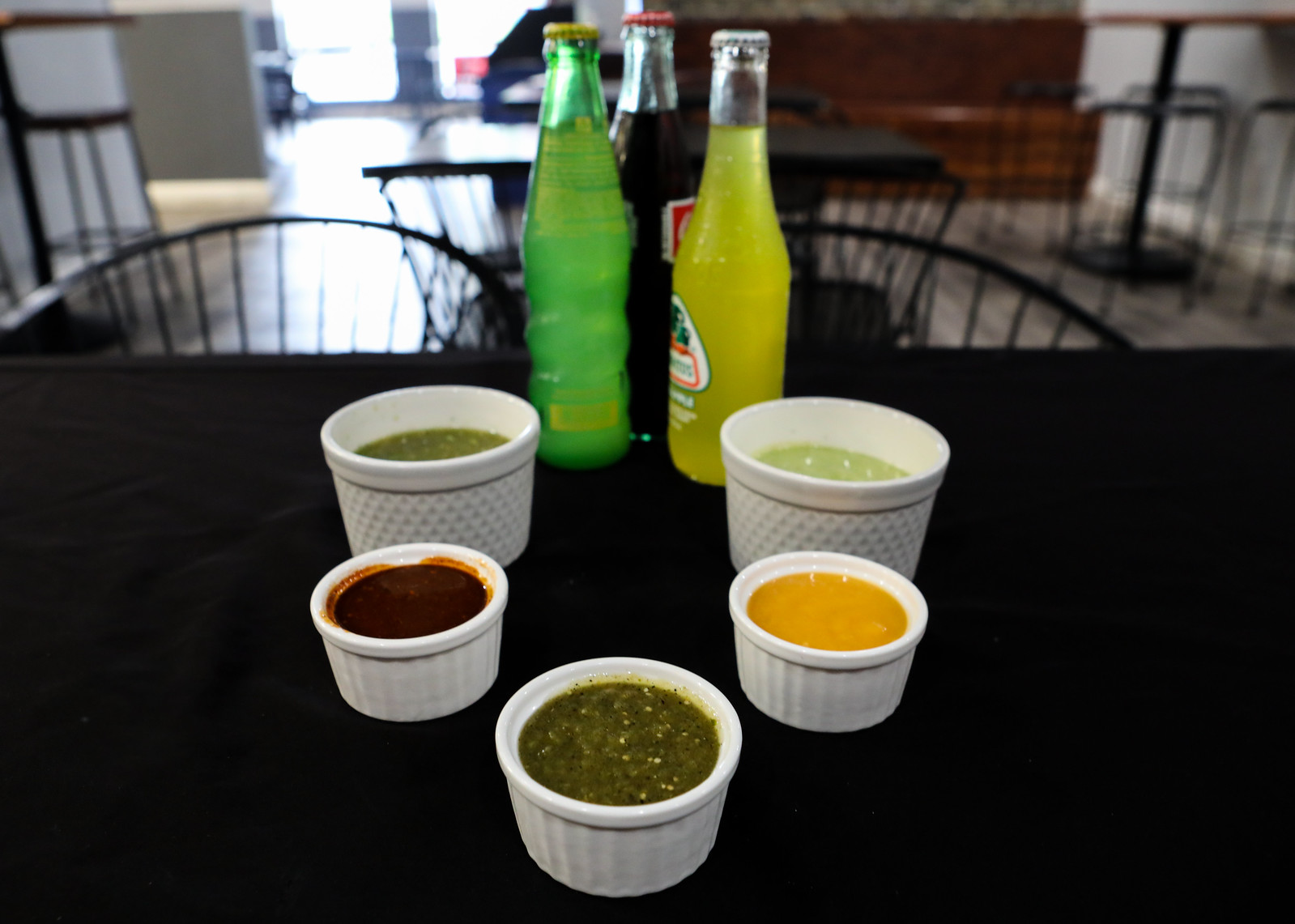The photograph captures a close-up of a neatly arranged assortment of dipping sauces and beverages on a black table, likely set in a Mexican restaurant. The focal point is the five ceramic ramekin cups positioned in a semi-circle. At the forefront is a small white cup with a green salsa. To its left is another white cup containing a dark red salsa, and behind it, a taller cup with a lighter green salsa, possibly an avocado-based sauce. On the right, we see a white cup with a vibrant orange puree, likely a smooth habanero salsa, and a taller white ramekin with a yellowish-green substance. 

In the background, three clear glass bottles of pop stand in a row. From left to right, there is a green bottle with a yellow liquid and a yellow cap, which appears to be a pineapple Jarritos, a dark amber bottle resembling Coca-Cola, and a greenish glass bottle with an unidentified light green liquid. The setting has a somewhat blurred background, revealing a bright, sunlit room with black tables and chairs, light gray flooring, and a hint of a dark brown wooden bench by the wall. Through the large windows, daylight filters in, casting a washed-out white hue across the scene.